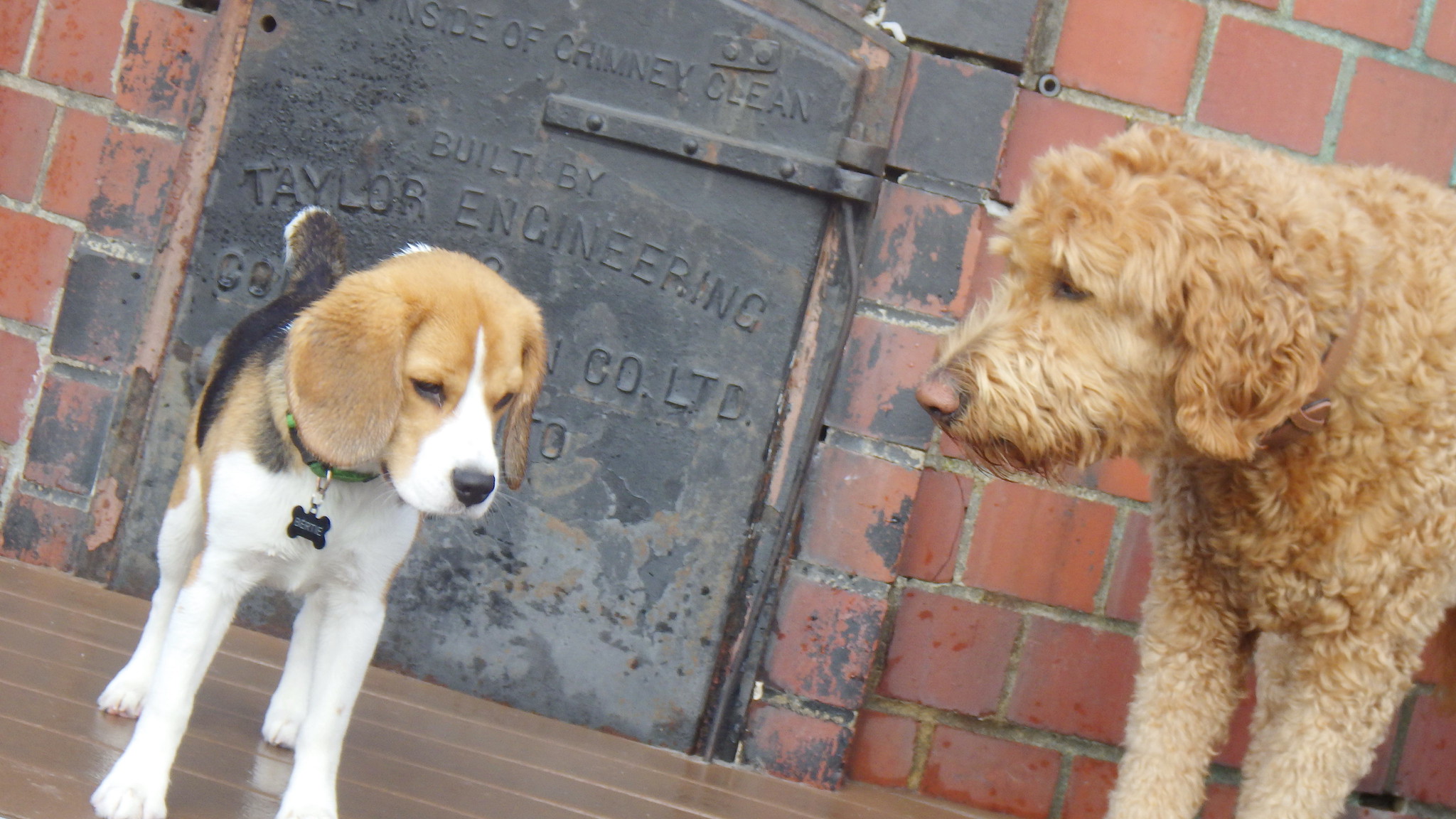In this image, we see two dogs standing on a shiny, wooden panel floor that features parallel lines. They are positioned in front of a red brick wall with a metal door that reads "Chimney Clean, Built by Taylor Engineering." The dog on the left is a beagle, identifiable by its distinctive tri-colored coat—mainly white with patches of brown and black—and has a black nose. It wears a green and black collar with a bone-shaped name tag that reads "Bertie" in white letters. The dog on the right is slightly larger, with curly, wiry fur of a reddish-beige color, resembling a wire-haired poodle. It has a light brown, tannish leather collar without a name tag. Both dogs appear to be focused on each other, with the larger dog looking at Bertie, and Bertie seemingly glancing down at the floor. There are no people in the image, making the interaction between the two dogs the focal point, further emphasized by the industrial backdrop with its distinct chimney door and brick wall.